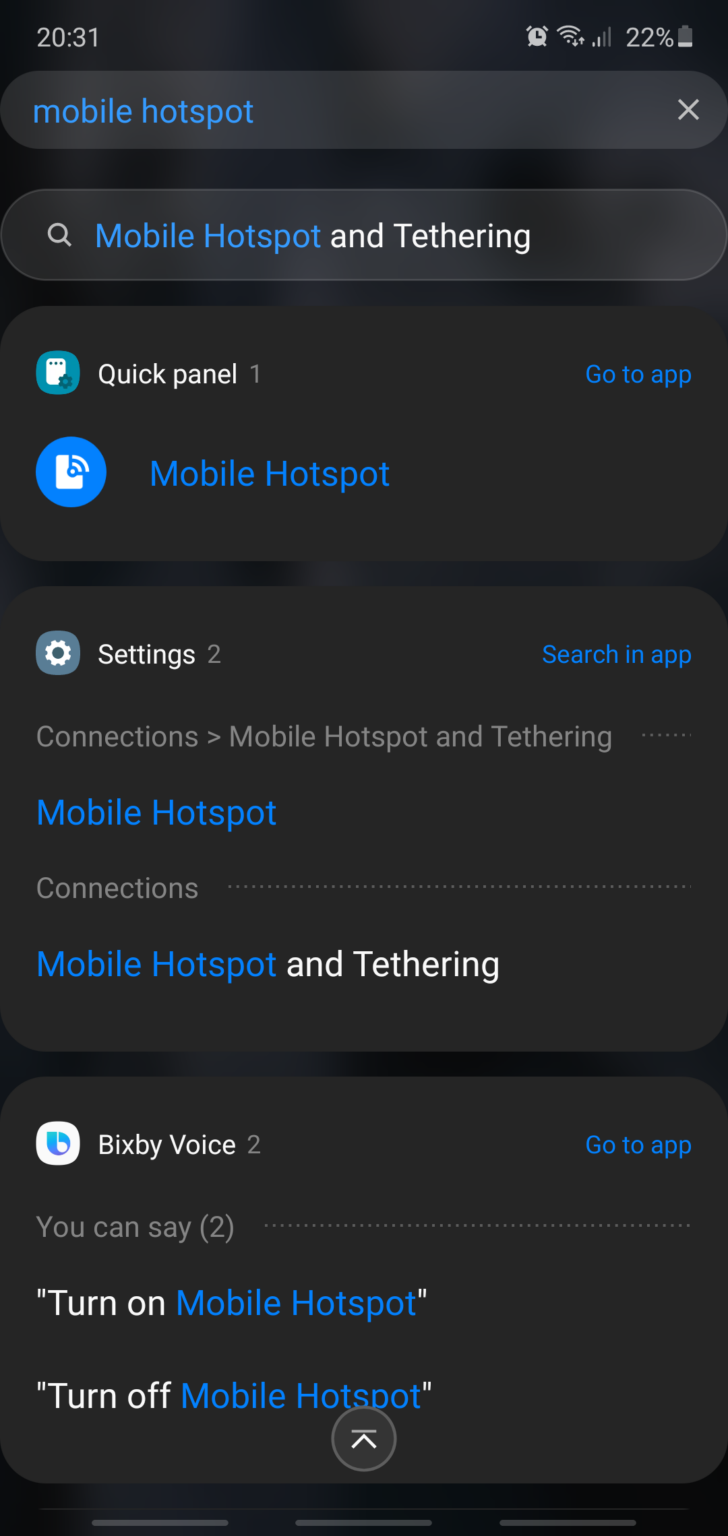In this image, we see a smartphone screen displaying the settings interface for a mobile hotspot. At the top of the screen, the status bar is visible, including indicators for the clock, signal strength, and battery level. The background of the interface is entirely black, with "Mobile Hotspot" prominently displayed in blue text at the top.

Below, a section labeled "Mobile Hotspot and Tethering" appears, where "Mobile Hotspot" is in blue and "tethering" is in white. This section also contains an option labeled "Quick panel" written in white, with "Mobile Hotspot" again listed in blue text adjacent to "Go to app" in blue on the far right.

Further down, there is another section labeled "Settings" in white text, next to which "Search in app" is shown in blue. Beneath "Settings," the subtitle "Connections" indicates the relevant settings category. This is followed by repeated mentions of "Mobile Hotspot and Tethering,” with "Mobile Hotspot" consistently highlighted in blue text and "tethering" in white.

Below the mention of connections, "Bixby Voice" is listed in white, alongside a blue "Go to app" link. At the very bottom of the screen, instructions are provided, stating, "You can say turn on mobile hotspot or turn off mobile hotspot."